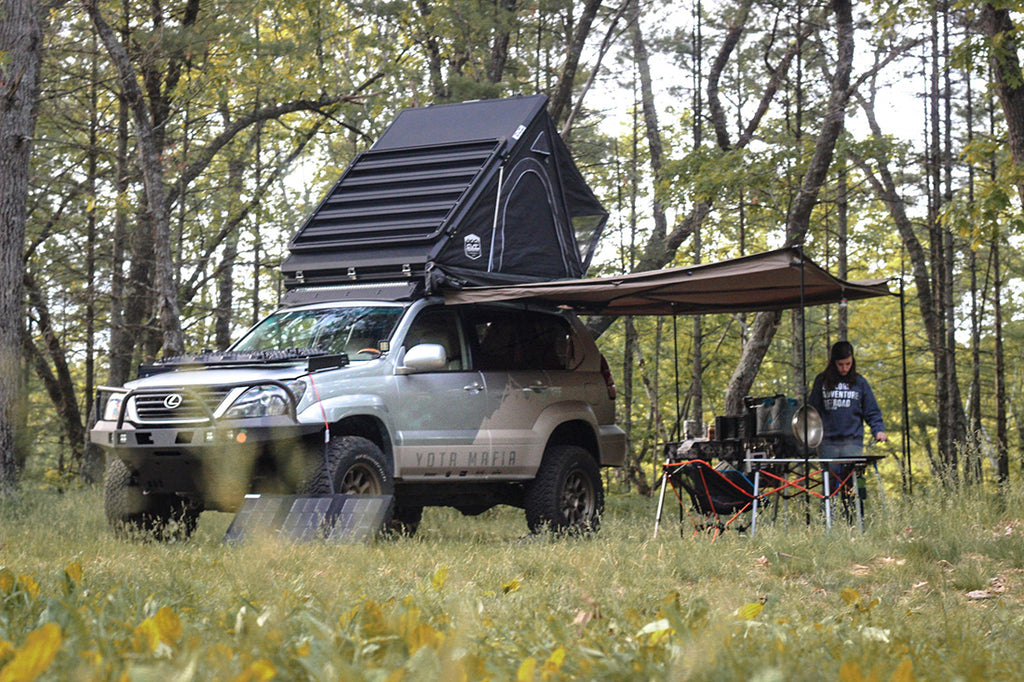In a lush, green clearing of a dense forest, a silver Lexus off-road SUV is stationed prominently. The SUV, with "Yoda Mafia" emblazoned on its side and equipped with rugged off-road tires and a distinct L Lexus grille, has a rooftop tent firmly attached, designed for sleeping accommodations. Attached to the vehicle is a brown awning supported by black poles, providing much-needed shade over a setup of outdoor equipment. Under the awning, a table laden with various items, including what appears to be cooking equipment and a pan, catches the eye. In the foreground, there is also a solar panel positioned near one of the wheels, suggesting an eco-friendly power setup.

A woman in a blue sweatshirt adorned with writing, and blue jeans is engaged in an activity at the table, possibly cooking. She stands focused on her task amidst the tall, green grass. The background reveals a dense cluster of trees, with sunlight breaking through the foliage and illuminating the scene, creating a serene and picturesque campsite.